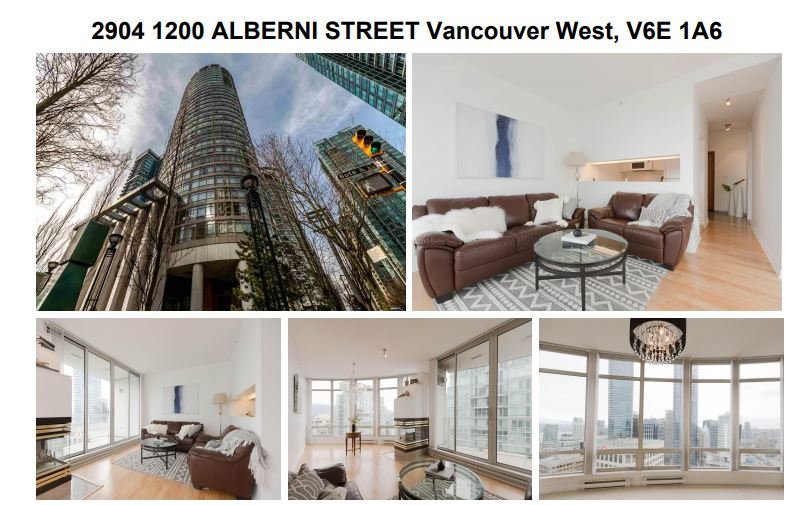Caption: "This is an informative collage showcasing a sophisticated apartment located at 2904-1200 Alberni Street, Vancouver West, V6E1A6. The layout consists of five images, with two positioned at the top and three at the bottom. The top-left image captures the striking exterior of the building, which appears to be approximately 20 stories tall, marked by its distinctive circular architecture and extensive use of glass. The photo is taken from the ground, looking up, and other towering skyscrapers are visible in the vicinity.

Adjacent to this, the top-right image offers a glimpse into the apartment's living area. It features elegant wood flooring adorned with a patterned area rug, and a sophisticated arrangement of furniture that includes a round glass table, coffee table, and a luxurious brown loveseat and matching sofa, presumably made of leather or vinyl. The walls are painted white, complemented by a minimalist artwork – a white canvas with a striking blue vertical stripe. The sofas are accentuated with white accessories such as comforters and pillows.

The bottom row of images adds more context to the living space. The leftmost image presents a wider perspective of the living room, emphasizing the expansive glass windows that the sofas face. The middle image extends this view, focusing from the sofa area towards an enclosed fireplace and additional floor-to-ceiling windows that bathe the space in natural light. The final image captures the impressive view from these windows, showcasing the curved architectural elements of the building and offering a panoramic outlook over the cityscape. A crystal-like chandelier hangs gracefully from the ceiling, adding a touch of elegance to the room."